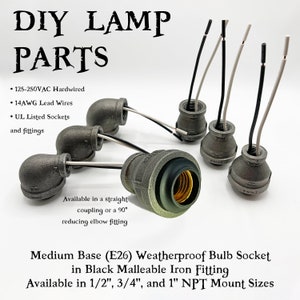This is an image illustrating DIY lamp parts, detailing their specifications and configurations. At the top, the text indicates "DIY lamp parts" followed by "125 to 250 voltage AC hardwired," "14 AWG lead wires," and "UL listed sockets and fittings." The image showcases a variety of fittings available in a street coupling or a 90-degree reducing elbow fitting. It features medium base, weatherproof E26 bulb sockets in black malleable iron, available in half-inch, three-quarter-inch, and one-inch NPT mount sizes. The lamp components are predominantly gray metal with visible wires extending from these sockets. The fittings and wires are arranged around a central fitting, and the overall appearance includes both metal and some rubber or plastic elements, with the fittings being primarily in a dull gray color, which serves as the focal point of the image.